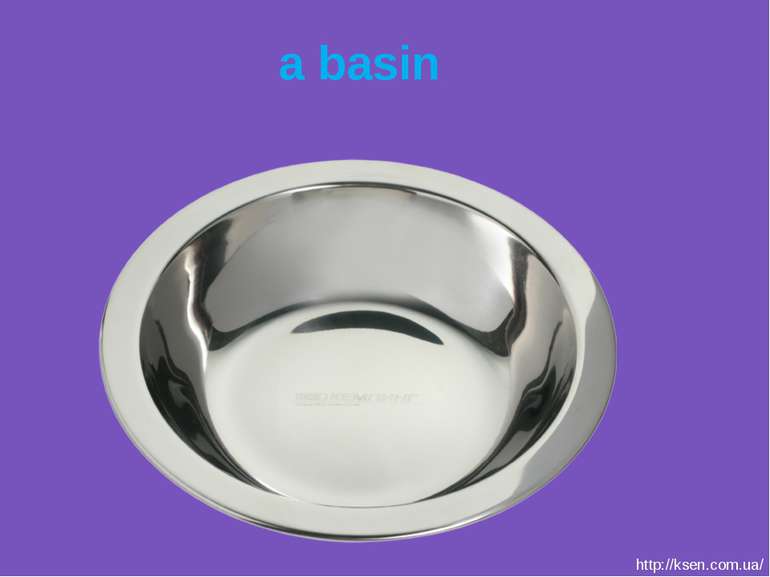The image features a solid silver basin prominently displayed in the center against a solid purple background. The basin is round, shiny, and resembles a dog bowl, complete with a lip around the edge and some black reflections on its surface. Above the basin, in lowercase light blue letters, is the text "a basin." The bottom right-hand corner of the image provides a white text URL, "http://ksen.com.ua," clearly visible against the purple background, presumably indicating the retailer's website. The basin itself is empty, and the brand stamp is visible at the bottom.